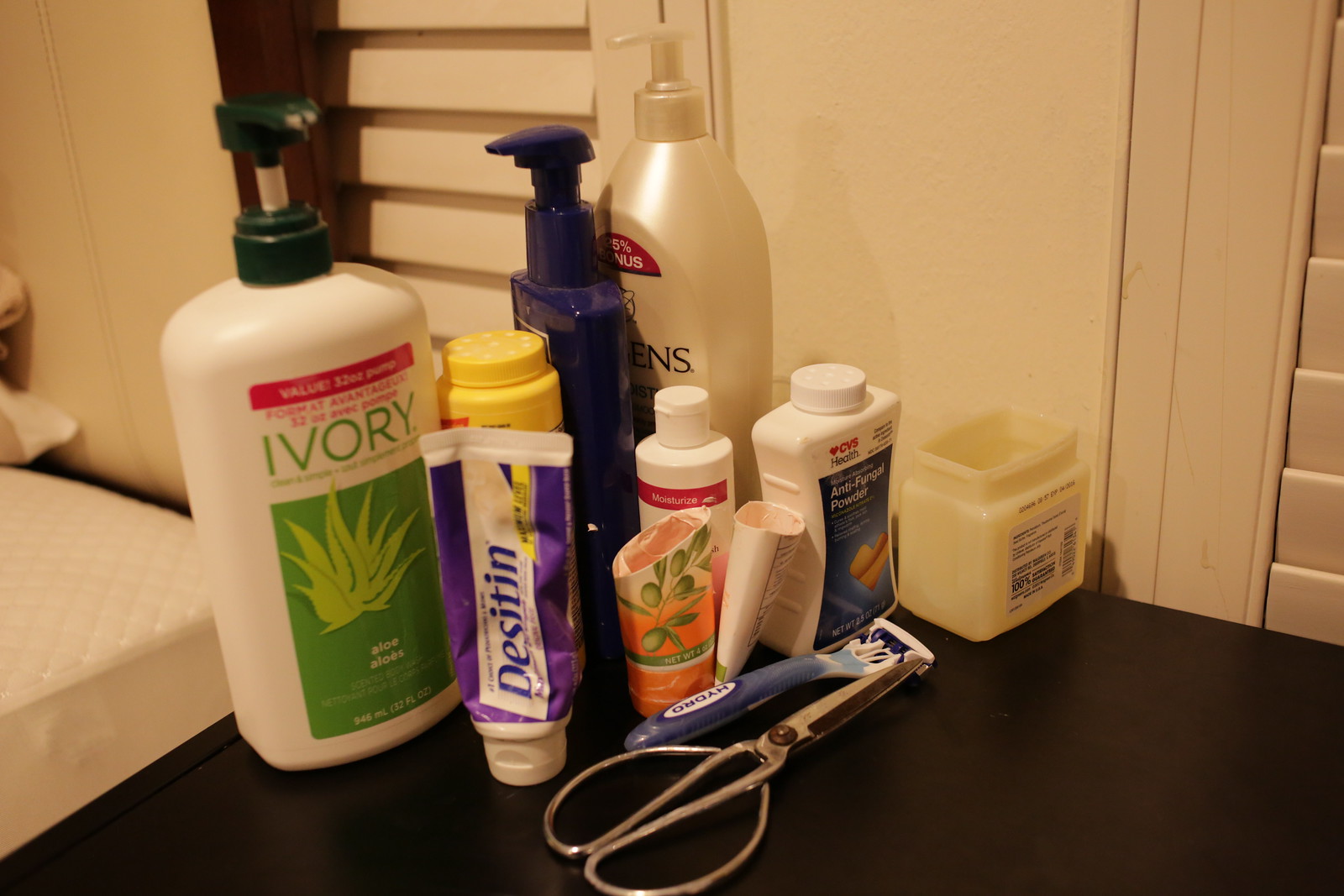In this photograph, taken in what appears to be a hotel room, various toiletries are meticulously arranged on a black desktop surface situated in the corner of a desk. The background features an off-white, light beige wall adorned with two vertical panels of shutters, potentially for windows or closets. On the left side of the image, slightly out of focus, is a bare mattress devoid of sheets, atop which are stacked a pillow and some blankets, barely visible at the edge of the photo.

Dominating the left side of the desktop is a large bottle of Ivory Aloe Lotion; its white body, green and red label, and green pump top make it easily identifiable. Adjacent to this is a small yellow bottle, its label obscured by a visually predominant squeeze tube of Desitin, sporting a blue, purple, and white label. Further to the right stands a blue lotion bottle equipped with a pump top, followed by another pump-topped, ivory-colored bottle of Jergens lotion.

In the foreground, a variety of smaller items lie arranged. A squeeze tube, which has been cut open halfway down, rests open beside it. There is also a bottle of antifungal powder from CVS Health, an open tub of Vaseline, a disposable blue razor blade, and a pair of silver metal scissors with metallic handles. Each item is clearly discernible, contributing to a detailed and comprehensive depiction of the scene.